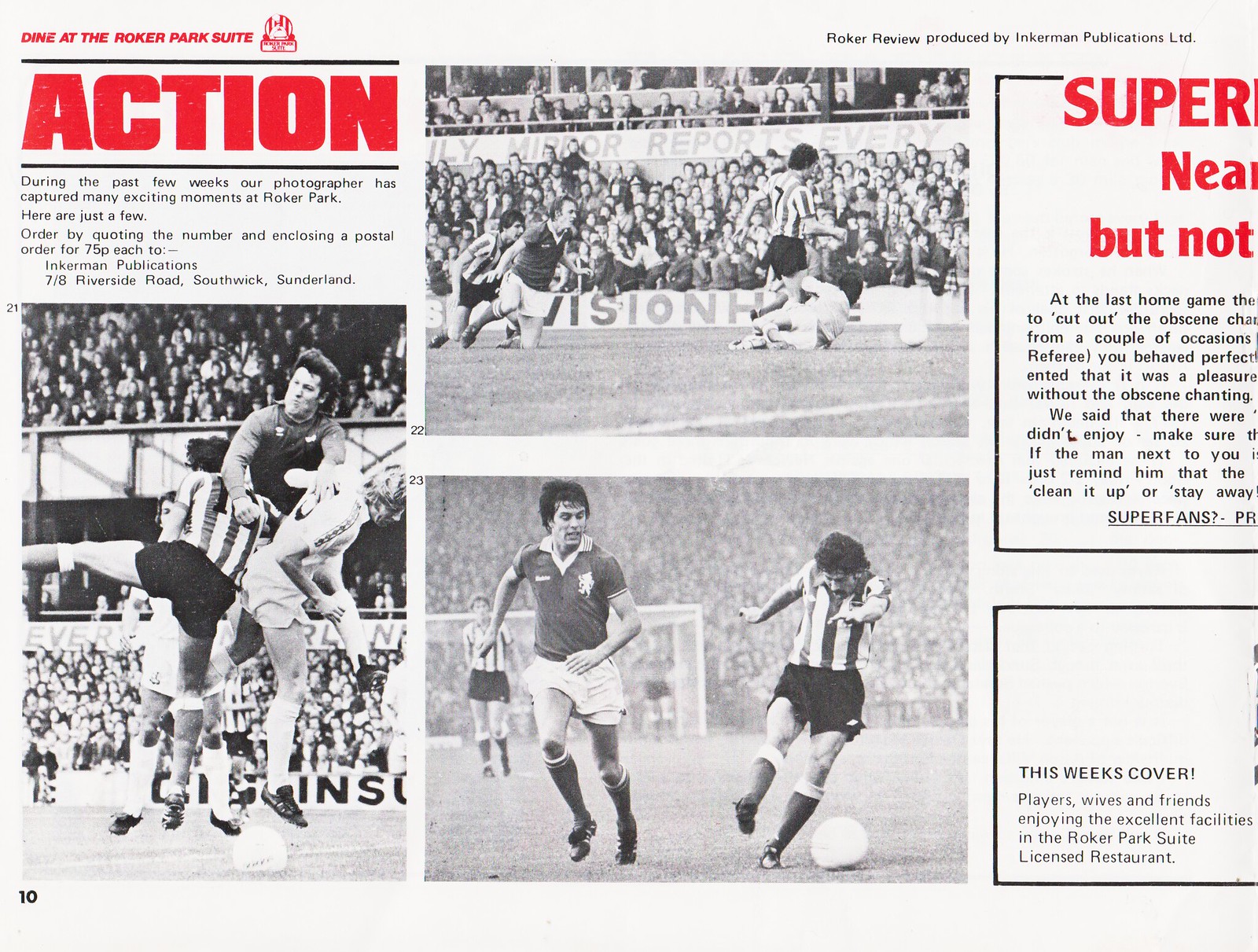This page from a sports magazine or periodical focuses on a series of black-and-white photographs capturing an exciting soccer match. At the top left of the page, the headline "Dine at the Roker Park Suite" is printed in red, followed by the bold red word "Action." Below, a paragraph reads: "During the past few weeks, our photographer has captured many exciting moments at Roker Park. Here are just a few." This text is accompanied by details on how to order these photos.

Dominating the central portion of the page are two photographs. The top photo shows soccer players running across the field in front of a stadium, while the bottom image offers a close-up of two players competing for the ball. On the left side, another image features four players jumping and colliding in mid-air, showcasing the game's intensity.

The right column contains more text, starting with the cut-off red letters "Super NEA" and "But Not." The article here is incomplete due to the page being cut off. Below this, a boxed section talks about "this week's cover," mentioning "players' wives and friends enjoying the excellent facilities in the Roker Park suite licensed restaurant,” but the image itself is not visible.

The page number, 10, is printed in the bottom left corner, and at the top right, the header "Roker Review produced by Inkerman Increment publication" indicates the source of the content. The combination of dynamic imagery and engaging descriptions emphasizes the excitement and atmosphere at Roker Park over the past few weeks.